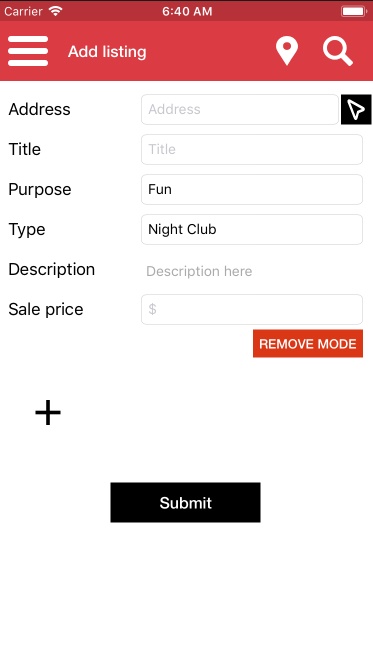The image is a screenshot of a form, divided into two main sections: a red upper section and a white lower section. The red section at the top contains the following elements: 

- On the upper left, the word "Carrier."
- In the upper center, the numerical value "640 AM."
- On the upper right, a fully charged battery icon.
- Below the battery icon, three horizontal white lines stacked on top of each other.

Beneath these elements, still in the red section, the text "Add Listing" appears in white, followed by a location icon and a search icon, both also in white.

The white section of the form contains fields for inputting various details:

- "Address" on the left, with a corresponding field on the right for entering the address.
- "Title" on the left, with a corresponding field on the right for entering the title.
- "Purpose" on the left, with the word "Fun" typed in the corresponding field on the right.
- "Type" on the left, with the word "Nightclub" typed in the corresponding field on the right.
- "Description" on the left, with the placeholder text "Description here" in gray in the corresponding field on the right, but nothing typed in.
- "Sale Price" on the left, with an empty space on the right for entering the price.

Below these fields, there is a red button labeled "Remove Mode," and to the left beneath it, a large plus sign. At the very bottom, there is a black button with the text "Submit" in white.

This form appears to be designed for creating a new listing, specifically suggesting a fun nightclub, with the option to submit the listing at the end. The app or platform to which this form will be submitted is not identified in the image.